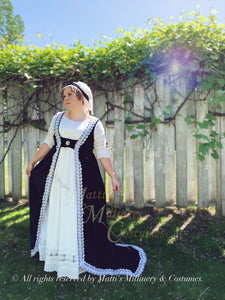This photograph, captured in daylight, showcases a young Caucasian woman standing outdoors against a clear blue sky. She is attired in a colonial or medieval-style costume featuring a long, white dress with three-quarter length sleeves. Over the dress, she dons a black, floor-length vest that drapes down her sides and trails slightly behind her. The vest is adorned with white trim along its edges. Her attire is completed by a white bonnet held in place by a black band, giving her a distinct old-fashioned look.

The woman stands on green grass in front of a tall, gray wooden picket fence, which is covered in vibrant green leaves and brown stems draping over its top. Her hands rest at her sides, and she gazes slightly upwards to the left. At the bottom of the image, there is a partially blurred inscription mentioning "all rights reserved," hinting at an advertisement logo for a costume store. Despite the low quality and small size of the image, the overall scene evokes a nostalgic, vintage ambiance.